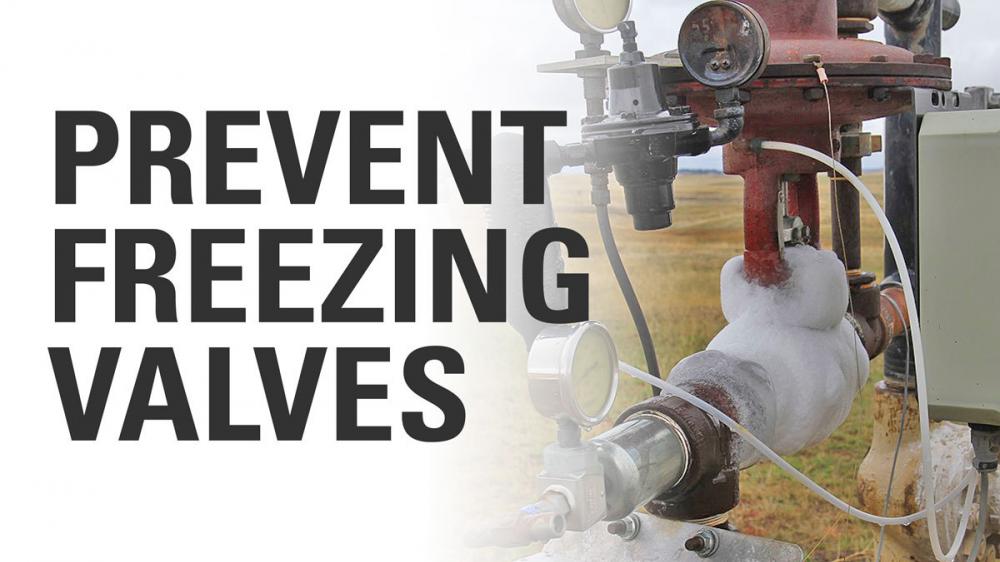The image is a poster designed to highlight a solution for preventing freezing in outdoor valves. On the left half of the poster, large black block letters on a white background read "Prevent Freezing Valves." The right half features a detailed photograph of what appears to be an insulated valve system, possibly used in agricultural or oil well equipment, situated in a field that might be meadowland or agricultural terrain.

The key component in the image is a large, red metal pump prominently displayed in the middle of the scene. Various pressure dials and gauges can be seen attached to this pump, along with several pipes, some of which are covered in thick white insulating foam that gives the appearance of packed snow. This foam likely serves as an insulating sock to prevent the valves from freezing.

Beneath the red pump is additional piping, and there’s also an electrical box to the right side of the photograph, indicating that the setup includes some electrical components. The close-up nature of the shot emphasizes the intricate details of the valve and its protective measures, showcasing the effectiveness of the insulation in keeping the mechanisms operational despite outdoor conditions.